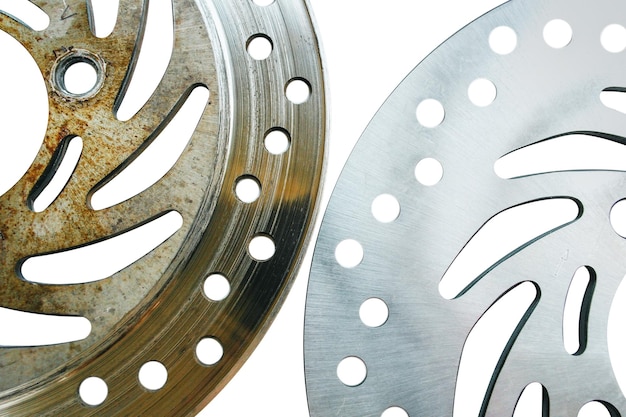The image depicts two metallic discs, likely automotive brake discs, positioned side by side. The disc on the left is coated with rust, distinguished by its darker hue and an orange tint suggestive of corrosion. This disc features numerous small, punched-out circles toward the perimeter and elongated, oval-like cutouts near the center. In contrast, the disc on the right appears cleaner and new, showcasing a shiny silver surface. Like the left disc, it also has circular perforations around the edge and similar oval cutouts at the center. The background is a plain white, enhancing the visibility and shine of both discs, emphasizing their contrasting conditions.